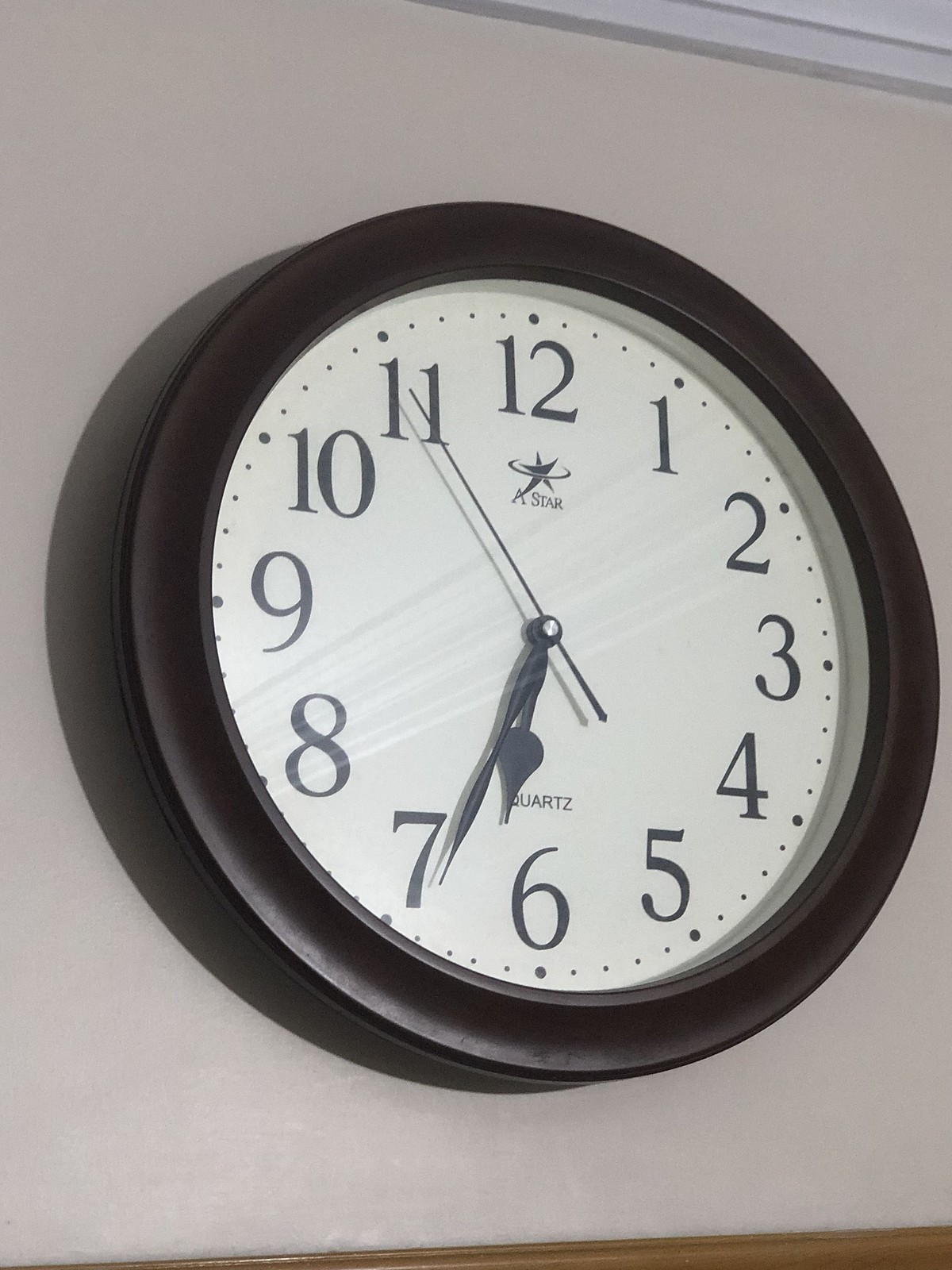The image showcases a close-up of a wall-mounted clock with a thick, black frame made of either metal or glossy plastic, reflecting some light. The clock rests against a white wall, with a wooden brown element at the bottom, possibly an elevated baseboard or a shelf. The time displayed is just after 6:30. The white clock face features black lettering, with the word "Quartz" and the brand name "ASTAR" accompanied by a small logo.